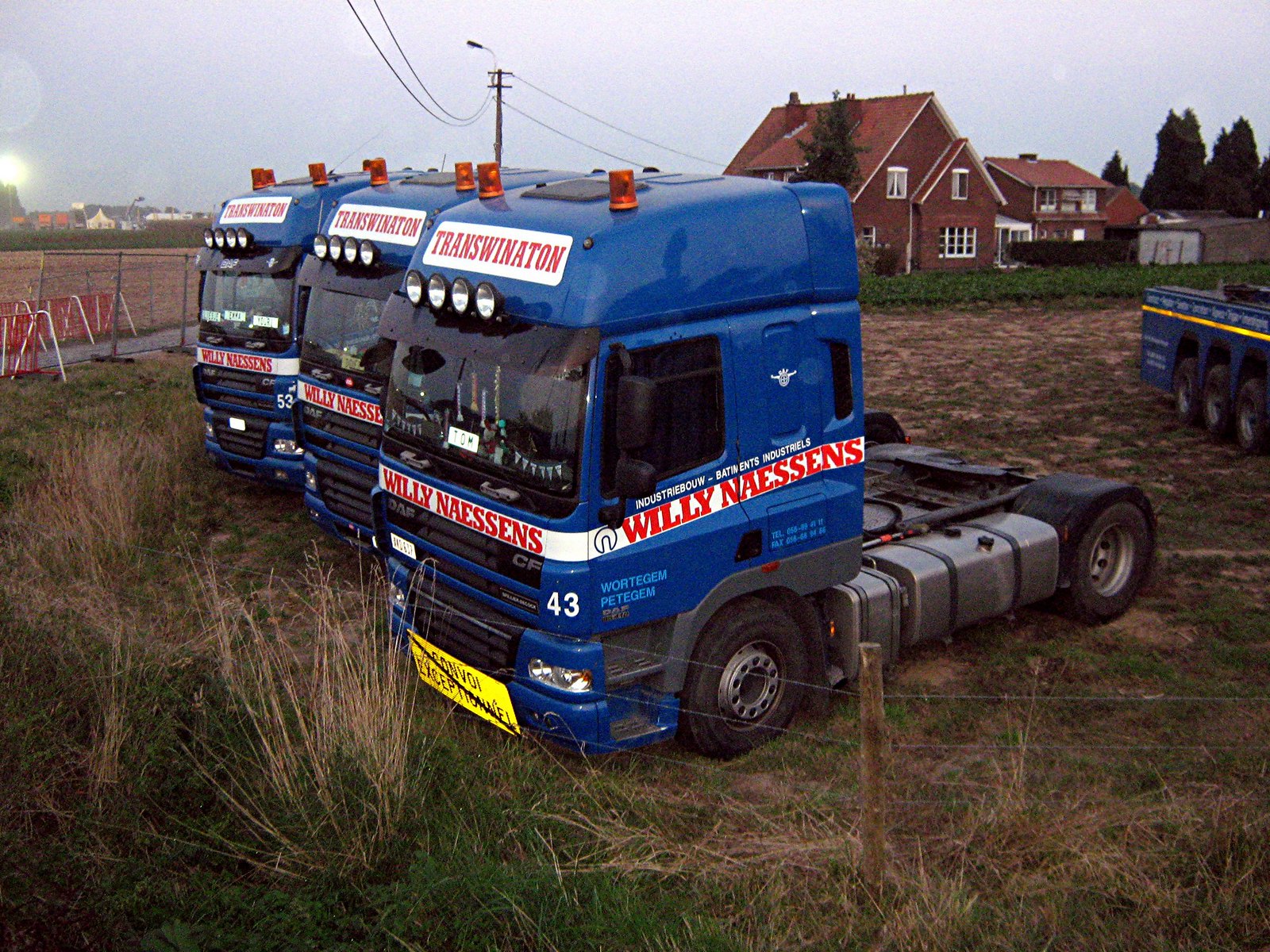In this image, three blue European semi-truck cabs are parked in a brown, grassy field that needs more water, alongside a fourth truck cab. Each truck features red text against a white background, with "Transwiniton" above the windshield and "Willie Nascence" below. The scene appears to be captured on a somewhat overcast day, in Europe. In the right part of the image, a blue trailer, positioned perpendicularly, reveals three visible wheels. The field is enclosed by a fence, with another fence running parallel to a road or pathway that leads to additional grassy fields. A backdrop of residential areas includes a prominent brick house with a tree nearby, and more houses, some from a distant housing subdivision, under a web of electric wires.